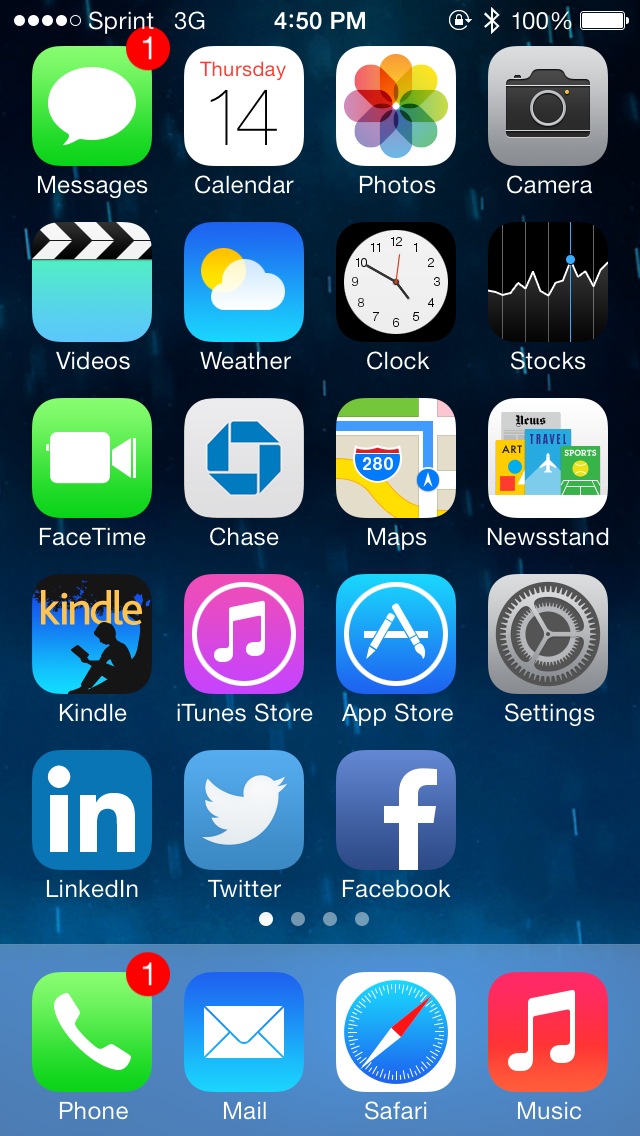This image showcases the home screen of an iPhone with a detailed and organized display of various app icons and status information. In the upper right-hand corner, there is a battery indicator at 100%, next to symbols for Bluetooth and a locked orientation icon encased in a circle. On the upper left, four filled dots and one empty dot signify the home screen page, alongside the text "Sprint 3G." At the top center, the time is displayed as 4:50 PM.

The first row of app icons includes:
1. **Messages**: A green and white speech bubble with a red notification badge displaying the number '1.'
2. **Calendar**: Showing "Thursday the 14th."
3. **Photos**: Featuring a multicolored flower.
4. **Camera**: Depicting a camera icon.

The second row consists of:
1. **Videos**: An app for video playback.
2. **Weather**: A weather forecast app.
3. **Clock**: For timekeeping.
4. **Stocks**: Financial market updates.

The third row has:
1. **FaceTime**: A green and white video call icon.
2. **Chase**: A gray and blue icon for Chase Bank.
3. **Maps**: An Apple Maps icon depicting a map.
4. **Newsstand**: Featuring images of books and magazines.

The fourth row includes:
1. **Kindle**: Marked in orange with a silhouette of a person reading.
2. **iTunes Store**: A purple and white shopping bag icon.
3. **App Store**: A blue and white icon for downloading apps.
4. **Settings**: A silver gear icon.

Additionally, there are icons for:
- **LinkedIn**: Displaying the "IN" logo against a blue background.
- **Twitter**: Represented by a white bird on a blue background.
- **Facebook**: Featuring a white "F" on a blue background.

Finally, the bottom row, within the dock, contains:
1. **Phone**: A green and white phone icon.
2. **Mail**: An envelope against a blue background.
3. **Safari**: A compass icon in red, white, and blue.
4. **Music**: A red icon with a white musical note.

The image provides a clear snapshot of an individual's iPhone interface, capturing not only the app icons and their respective positions but also detailed status information available at the top of the screen.